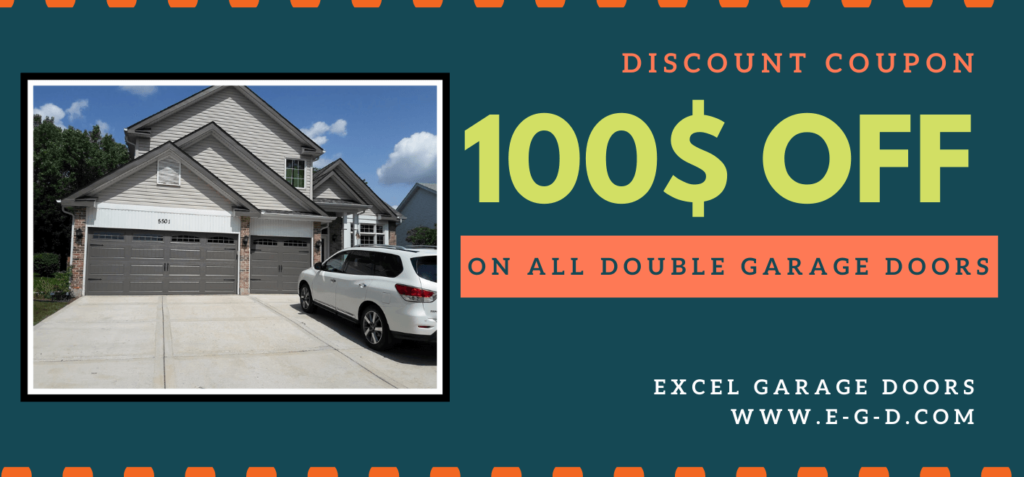This advertisement features a visually appealing, ticket-shaped coupon set against a dark blue-green background with orange borders along the top and bottom edges. On the left side of the ad, there is an embedded image of a two-story house, highlighting its two garages, a spacious paved driveway, and a white estate car parked in front. The right side of the image prominently displays digital text offering a "Discount Coupon: $100 off on all double garage doors," clearly indicating the promotion. The company name, XL Garage Doors, is mentioned along with their web address, www.e-g-d.com, guiding potential customers to their website.